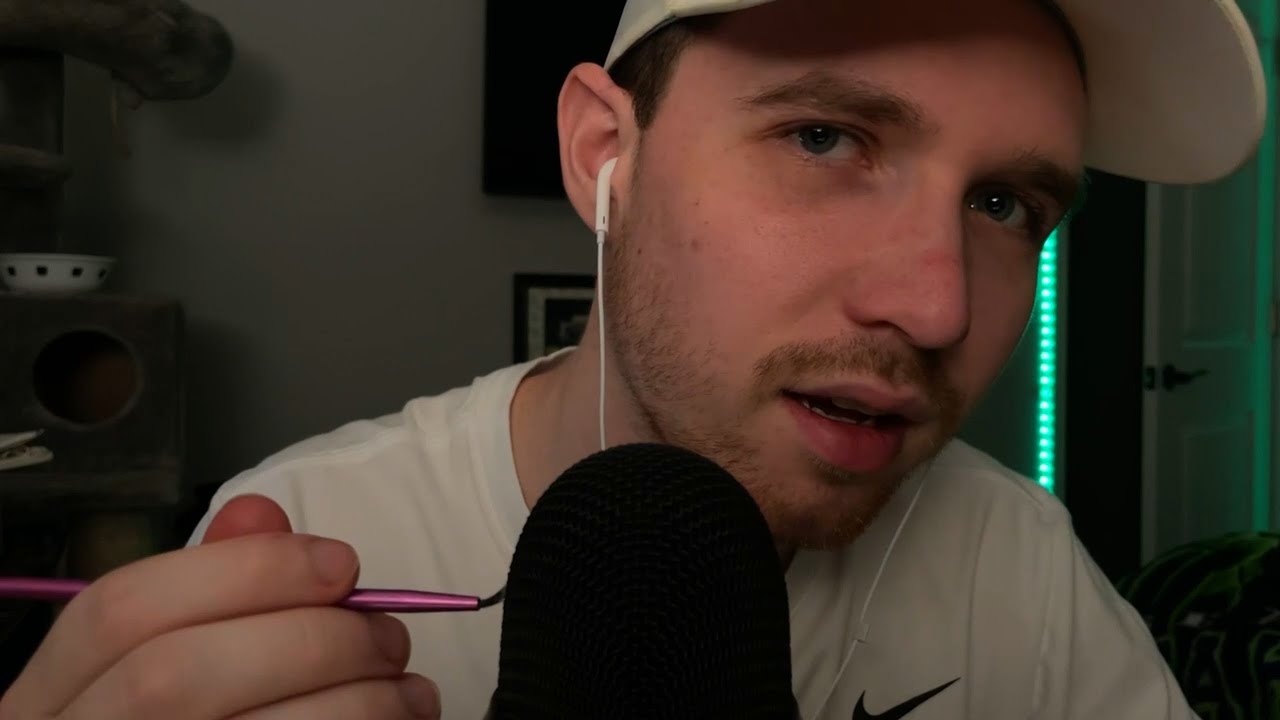A young man, likely in his mid-20s, is featured in this close-up shot. He is seated in what appears to be his bedroom; the partially open drawer and blinds, along with a few pictures and miscellaneous items stacked on the left, suggest a casual, home setting. He sports a bit of facial hair, including a noticeable mustache, and wears white earphones. His white ball cap and white T-shirt with a black Nike swoosh add to his casual appearance. He holds a dental instrument – a metal scraper-like tool – between his right index finger and thumb. There's a black object positioned in front of him, possibly a microphone or a censor, adding a layer of intrigue and ambiguity to the scene. His head is slightly tilted to the left, focusing intently on something off-screen.